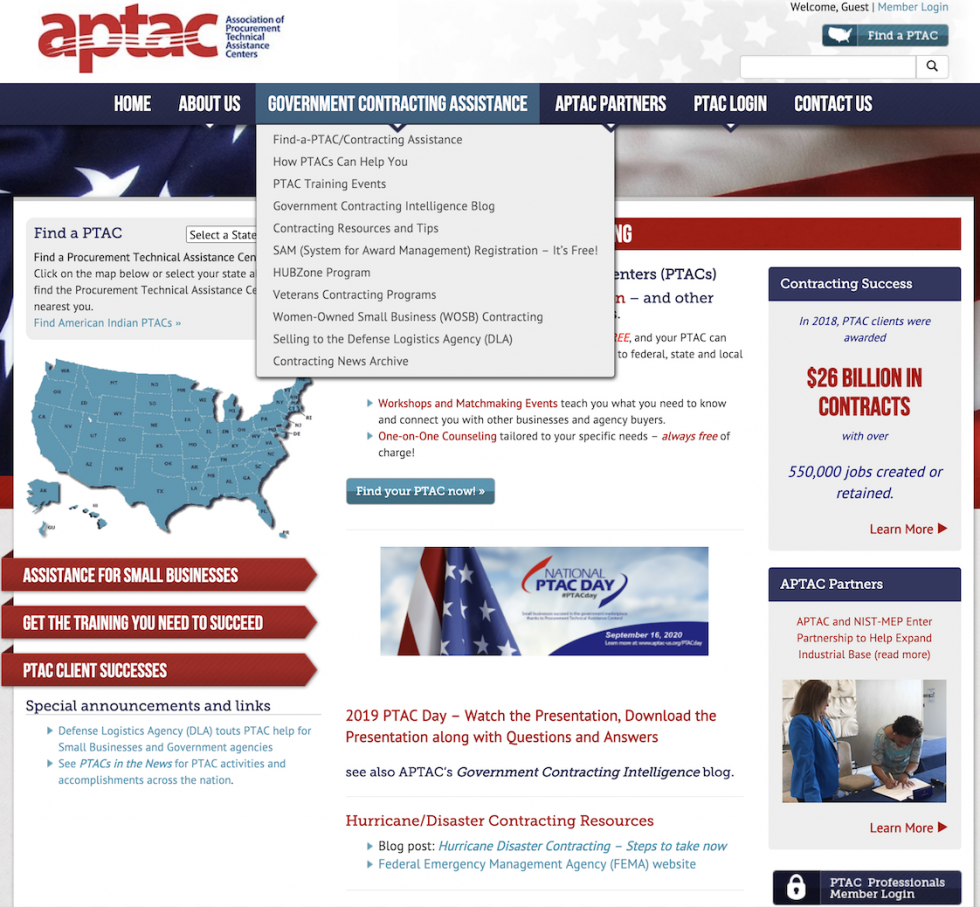The image showcases the desktop homepage of the APTAC (Association of Procurement Technical Assistance Centers) website. The APTAC logo, in small red letters, is prominently located at the top left, accompanied by the full association name in small blue letters to the right. The background features a faint image of stars from the USA flag, adding a patriotic touch to the header.

In the top right corner, the website greets visitors with "Welcome Guest" in small black font, followed by a "Member Login" link in small blue font. Below these, there's a blue button adorned with a map of the United States to the left, next to the text "Find APTAC." The bottom right corner of the header includes a search bar with a magnifying glass icon for easy navigation.

Directly beneath the header, a blue border spans the width of the page, delineating the navigation menu. The menu lists several categories: Home, About Us, Government Contracting Assistance, APTAC Partners, PTAC Login, and Contact Us. The 'Government Contracting Assistance' category is highlighted in light blue, indicating it has been selected. Expanding from this selection, a vertical dropdown box appears with a list of subcategories: 'Find a PTAC', 'Contracting Assistance', 'How PTACs Can Help You', 'PTAC Training Events', and more.

In the background, a section on the left features another 'Find a PTAC' dropdown box allowing users to select a state. Adjacent to this is a blue-colored map of the USA. Below this, a banner promotes assistance for small businesses, offering training to aid in their success, and highlights PTAC client achievements.

Lastly, in the bottom right of the page, a white lock icon is accompanied by the text "PTAC Professionals Members Login," providing access for PTAC members to securely log in.